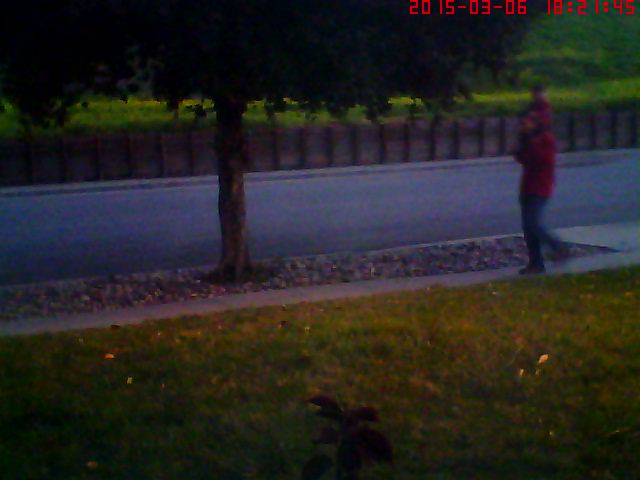The image, which is somewhat blurry and may be from a door camera or similar device, was taken on March 6, 2015, at 18:21:45. It shows an outdoor setting with a manicured patch of green grass in the foreground, covered sporadically with reddish-pink leaves. This grass leads up to a concrete gray sidewalk. On the sidewalk, a man is walking while carrying a child on his shoulders; the man is wearing a reddish coat, blue jeans, and medium brown shoes, and has dark hair. The child's hands are resting on the man's head, and the child is dressed in a similarly colored reddish coat over what appears to be pinkish or purple clothing. Past the sidewalk lies a small gravel area with a solitary tree, which has a circle of gray stones around it and is full of green leaves. Beyond this area is a gray asphalt road, which is bordered by a grayish-brown fence with evenly spaced posts. In the distant background, there is a large green field stretching out, possibly part of a hill, under ambient light. This scene is slightly out of focus, giving it a softened effect.